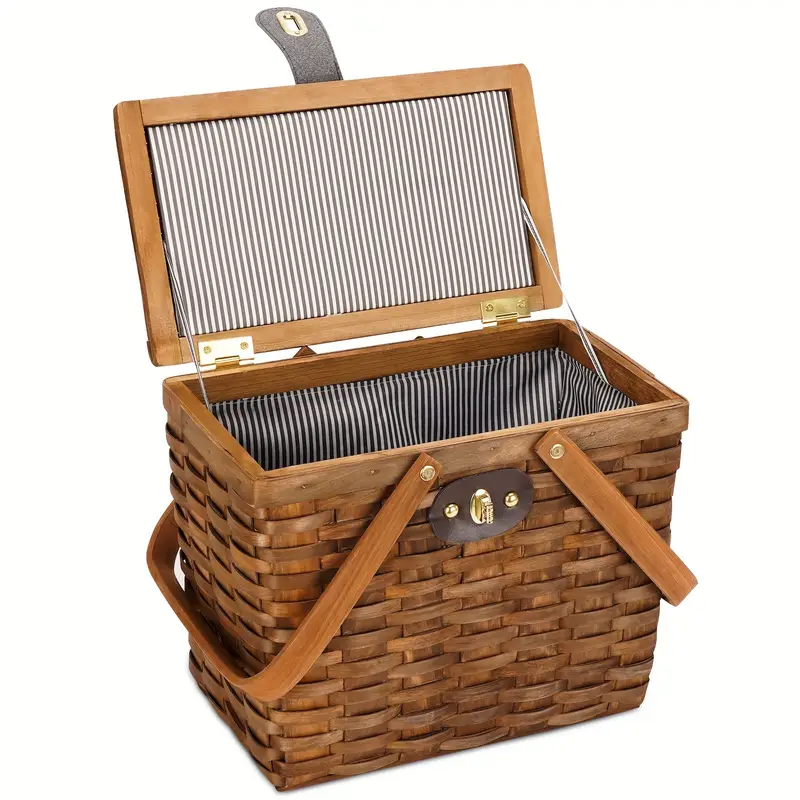The image showcases a tall, rectangular wicker picnic basket that is brown in color. Its open lid, held by brass-colored hinges and two metal rods, reveals an interior lined with alternating blue and white vertical stripes. The lid features the same cloth material and can be securely fastened by a bronze-gold latch mechanism, complete with a small leather flap. The basket boasts two wooden handles on each side, which can be flipped up for easy carrying when the lid is closed.